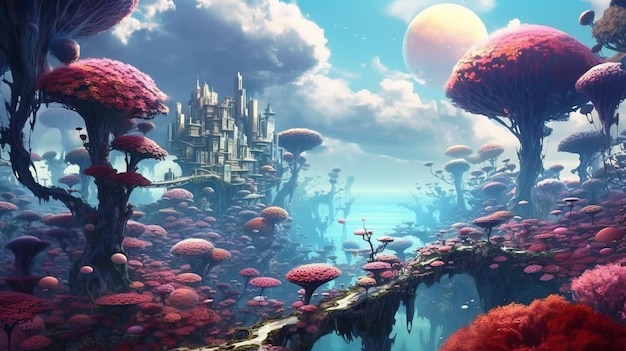The image is a digital illustration or AI-generated artwork portraying an otherworldly, fantasy forest scene. It features a towering, multi-layered castle or fort in a grey or brown hue, situated on a steep island towards the left side of the image. Above the castle, dark, fluffy clouds loom, blending shades of grey and white. In the sky, a pale pink, spherical celestial body—either a moon or a planet—glows gently. 

Dominating the foreground, trees and plants shaped like mushrooms, with pink and red flowers and blood vessel-like trunks, create a surreal, vivid landscape. These mushroom-like structures vary in size, with some having flat tops composed of small, darker pink flowers. A natural stone bridge with a walking path extends from the lower left-hand corner, crossing to the lower right, reflecting in a dark blue body of water that occupies this section.

The entire scene exudes a bluish glow, enhancing its fantastical ambiance. The upper right quadrant showcases a blue sky with scattered white clouds, while darker storm clouds gather to the west, adding an element of mystery to the enchanting setting.